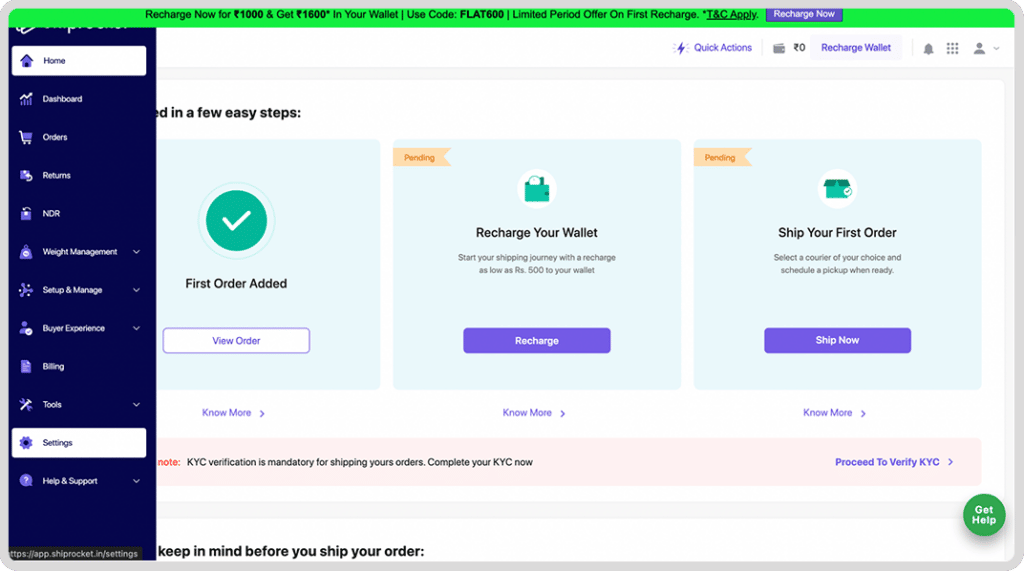The interface appears to be a dashboard for an e-commerce platform, potentially WooCommerce, though the specific platform is unclear due to a partially obscured logo. A prominent green notice at the top reads: "Recharge now for $1,000, get $1,600 on your wallet. Use code flat600, limited time offer for reverse free charge. Terms and conditions apply. Recharge now," accompanied by a purple button.

On the left side, there is a vertical, purple-colored navigation menu. The currently selected item is the "Home" button, highlighted in white. Other menu options include:
- Dashboard
- Orders
- Returns
- NCR (possibly)
- Weight Management
- Setup/Manage
- Buyer Experience
- Billing Tools
- Settings (also selected)
- Help and Support

On the main interface, the top section prompts the user to "Enter something in a few easy steps." There are three main action buttons:
1. **View Order:** Displayed with a green circle and a checkmark, indicating it's selected.
2. **Recharge:** Features an icon of a wallet and is pending action.
3. **Ship Now:** This is also pending action, featured just below the recharge button.

All buttons are purple in color. Beneath these options, there are additional buttons, including:
- **Proceed to Verify KYC**
- **Get Help** located in the lower right corner.

A note beneath these buttons reads: "KYC verification is mandatory for shipping your orders. Complete your KYC now."

Each section is well-defined with clear action items, despite the uncertainty around the platform's identity.